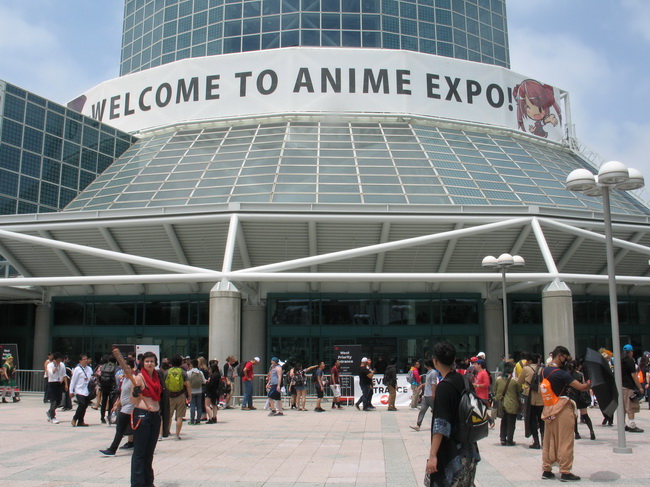This vibrant, mid-day scene captures the bustling exterior of an Expo Center, adorned with a striking architectural design predominant in glass and large cylindrical white pillars. Dominating the top of the building, a prominent banner emblazoned with "Welcome to Anime Expo" spans across, complete with an anime girl character illustration to the right. Below, the crowd of diverse adults, some in casual attire and others dressed as distinctive anime characters, animates the brick-floored expanse. Amongst the cosplayers, a notable woman on the left stands out in black pants and a red scarf, wielding a baseball bat. The complex array of hues in attendees' outfits includes blue, white, gray, dark blue, black, pink, orange, red, lime green, and light blue. The day is bright and sunny, highlighting the light poles and various signs that dot the scene, though the text on these signs remains unreadable. Throughout the central area and towards the building's entrance, guardrails manage the lines of attendees eager to enter the event unfolding within this creatively structured venue.